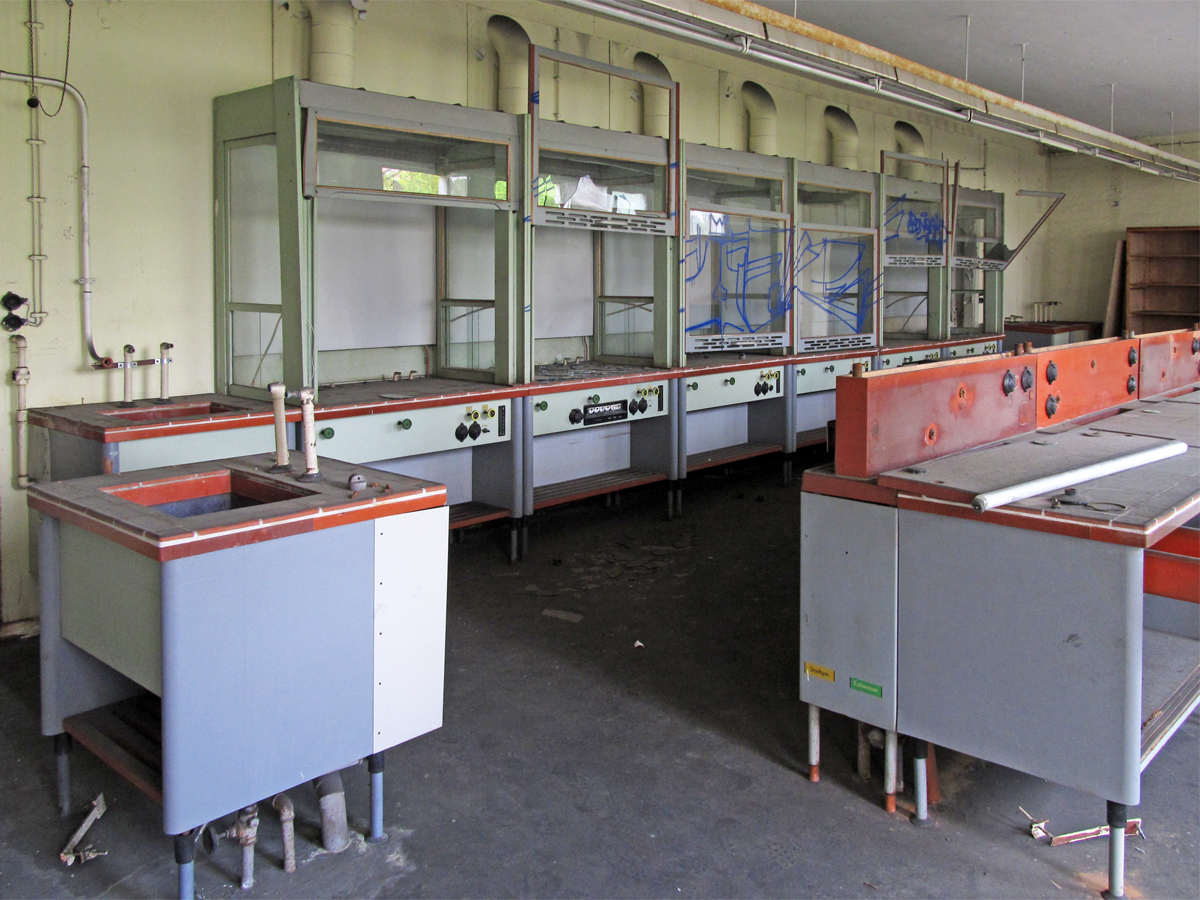The image depicts an industrial or laboratory workstation with an arrangement of six light blue machines, each featuring red tops, lined up against a light baby yellow wall. Above these machines, fluorescent lights run the length of the room, illuminating the scene with a stark brightness. On the left side of the image, there's a sink next to the machines, possibly accompanied by another sink towards the middle left. The floor appears to be gray, potentially concrete. Towards the front right, there are three tables with red countertops and metallic structures. These tables might be used for various tasks, distinguished by black knobs and holes on their surfaces. The left-hand side of the image also shows some light green cases with glass panels, housing blue cables or ribbons. Despite the overall orderly arrangement, the setting seems slightly neglected, indicated by rust on the light fixtures, enhancing the impression of an industrial or laboratory space that may not be in full active use. The photo gives an amateur feel, focusing clearly on all the elements without any text or additional description.